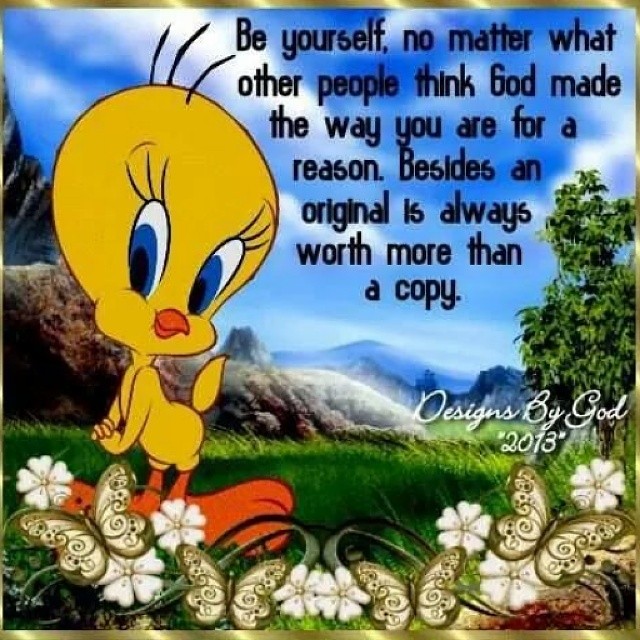The image showcases a vibrant cartoon outdoor scene with Tweety Bird prominently standing on a lush green grassy field. Tweety Bird, with his characteristic yellow feathers, blue eyes, and bright orange beak and feet, is positioned on the left-hand side. Surrounding him are white flowers and delicate beige butterflies. In the backdrop, there are scattered clouds in a bright blue sky, along with a leafy green tree on the right-hand side and a large boulder on the left-hand side. Further in the distance, a range of small hills and rolling mountains adds depth to the landscape. At the top of the image, in the upper right-hand corner, a quote reads: "Be yourself no matter what other people think. God made the way you are for a reason. Besides, an original is always worth more than a copy." This is followed by the text in cursive, "Designed by God 2013," located in the lower right-hand corner.